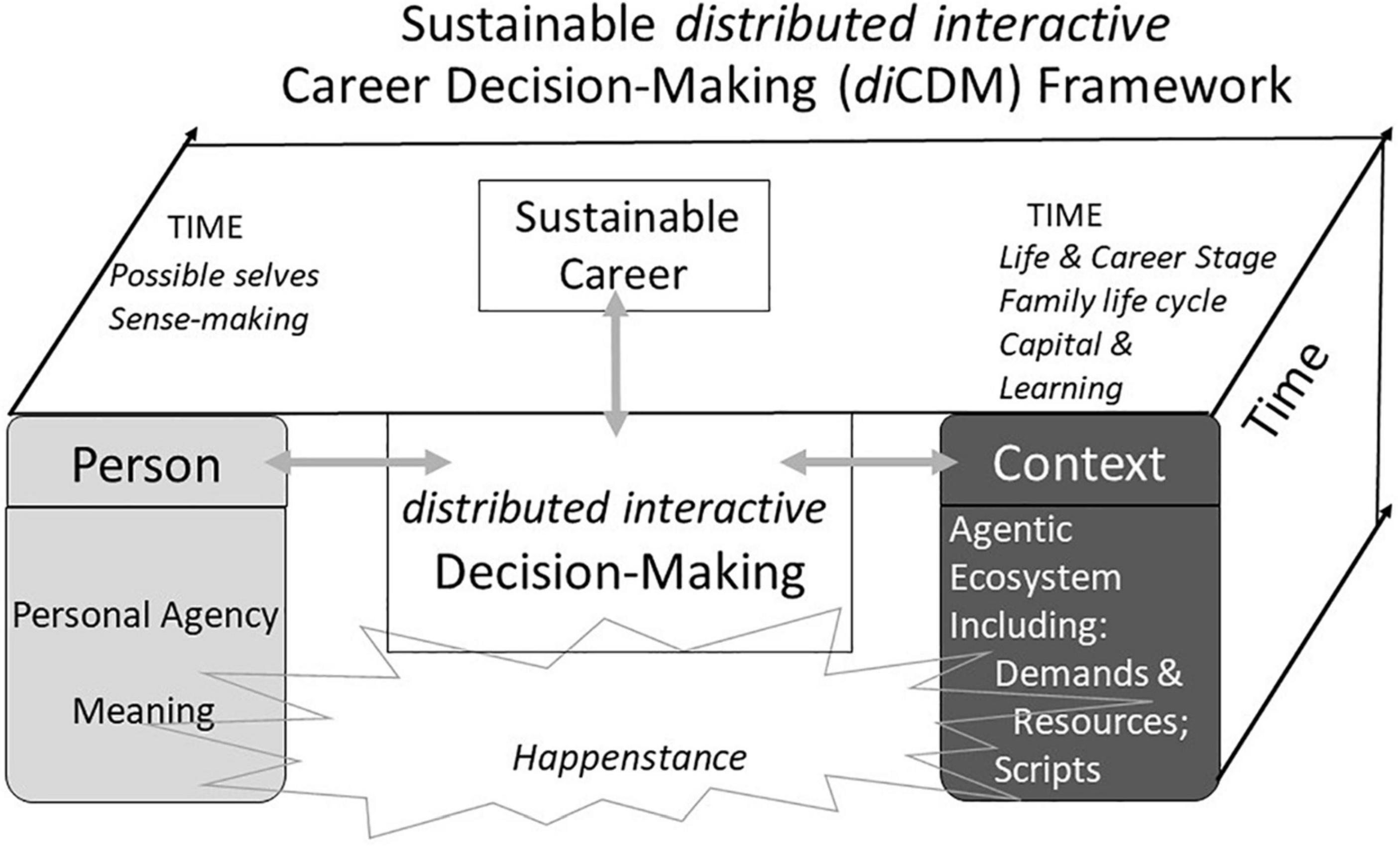**Detailed Caption for Diagram: Career Sustainable Distributed Interactive Career Decision-Making Framework**

The diagram titled "Career Sustainable Distributed Interactive Career Decision-Making Framework" (abbreviated as dICDM), visually represents the intricate dynamics involved in career decision-making. The framework is compartmentalized into various labeled sections interconnected with lines and arrows, highlighting the flow and influence of different elements.

On the left side of the diagram, a light gray box is labeled "Person." Below this, sub-labels such as "personal agency" and "meaning" indicate factors intrinsic to the individual that influence career decisions. 

Opposite to this, on the right side, a dark gray box is labeled "Context." This section delves deeper, with descriptors like "agentic ecosystem" which includes "demands and resources” as well as “scripts,” showing the external factors and environments that impact the decision-making process.

Additional factors illustrated in the diagram, variedly placed and interlinked throughout, include "happenstance," "time," and "sustainable career." These components suggest the various unpredictable events, temporal considerations, and long-term career sustainability all play significant roles in shaping career decisions.

Overall, the diagram encapsulates how personal and contextual elements synchronously interact to influence the career decision-making process, underscoring the complexity and distributed nature of this intricate framework.